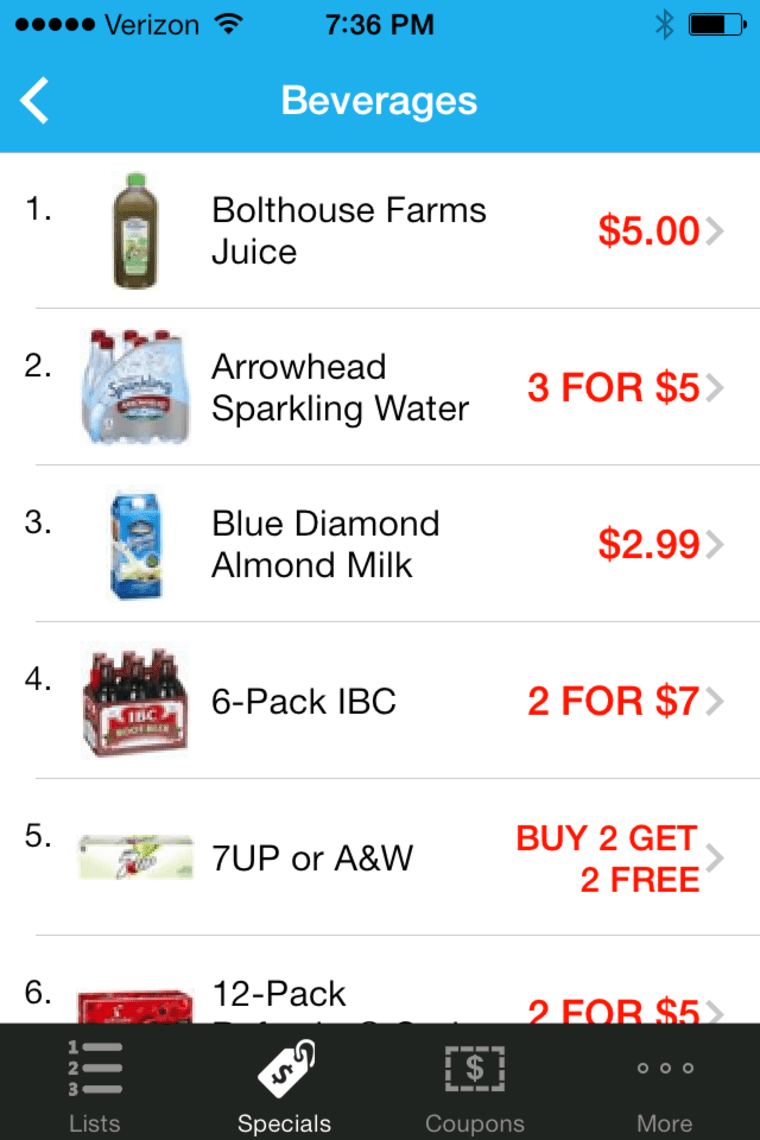At the top of the image, there is a blue rectangle with the text "5 days." In the upper left corner, six black dots are followed by the word "Verizon" in black font. Next to it, the Wi-Fi symbol shows 5 full bars. The central part of the top bar displays the time as 7:36 PM, while to the right, an icon indicates Bluetooth is off and the battery level is at 75%. 

Beneath this, a blue bar features the word "Beverages" in white font, accompanied by a white left-pointing arrow on the left side. Below this blue bar, a list is presented on a white background, delineated by faint black lines. Each item in the list is contained within small rectangles.

1. The first rectangle shows a picture of a bottle labeled "Bolthouse Farms Juice" with a red price tag reading "$5."
2. The second rectangle displays an image of a six-pack of Arrowhead Sparkling Water with a red label stating "3 for $5."
3. The third rectangle features "Blue Diamond Almond Milk" with a blue carton image and a red price tag marked "$2.99."
4. The fourth rectangle presents a six-pack of IBC with a red label stating "2 for $7."

This detailed layout efficiently provides a list of beverages with corresponding images and prices.